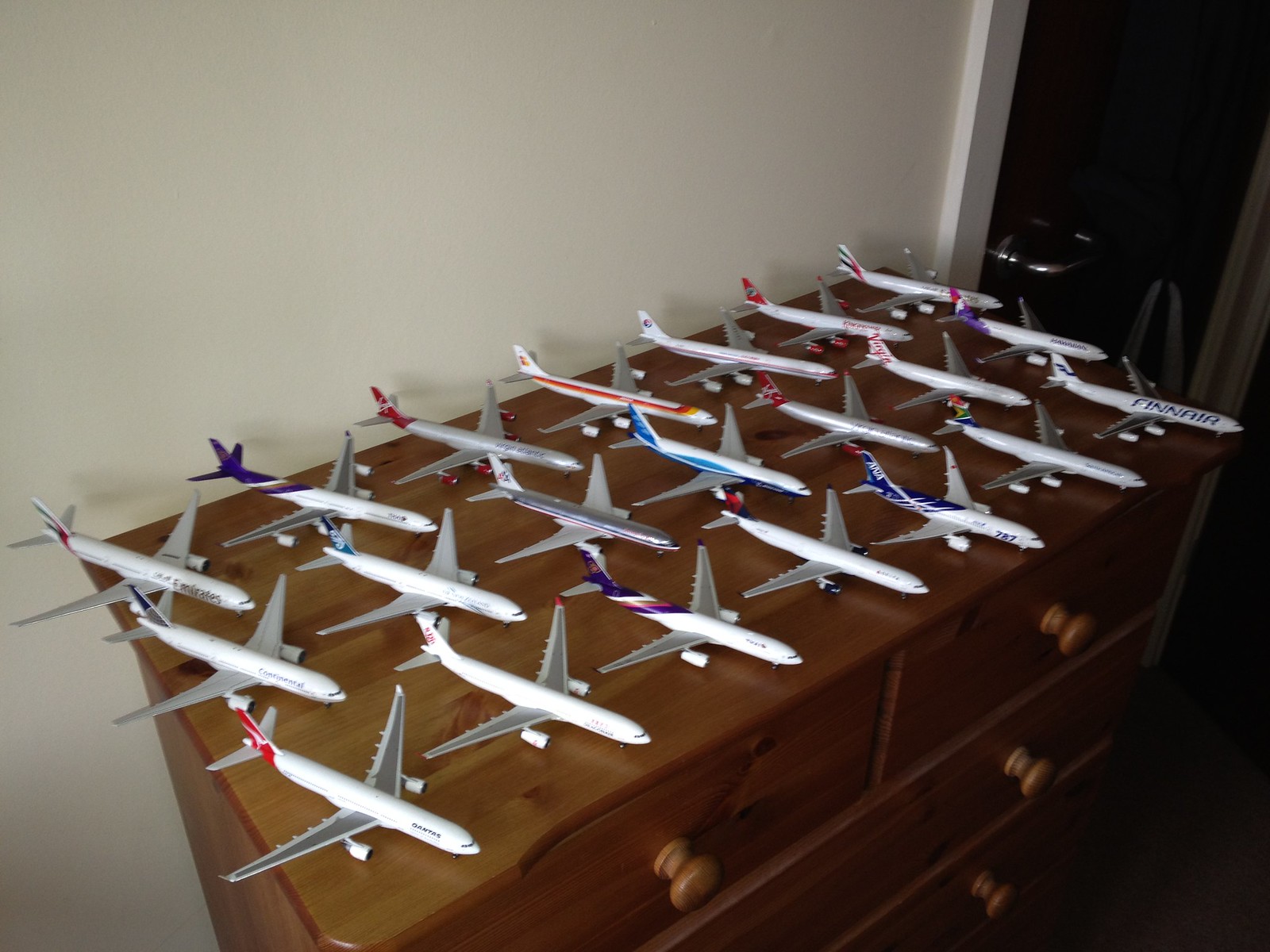This top-down photograph captures a wooden dresser adorned with a collection of 21 miniature passenger airplane models, meticulously arranged in three rows, each row comprising seven models. The dresser, constructed from brown wood, features prominent large brown knobs on its drawers. All the toy jets are positioned with their noses facing towards the front of the dresser. The airplanes are primarily white or grey, with some displaying colorful accents, such as blue or red tails, and one notable model with a red and orange stripe down its side. A specific model is marked with "Finna Air." The backdrop consists of a white wall with a black door situated in a shaded corner, which has a silver metal handle.